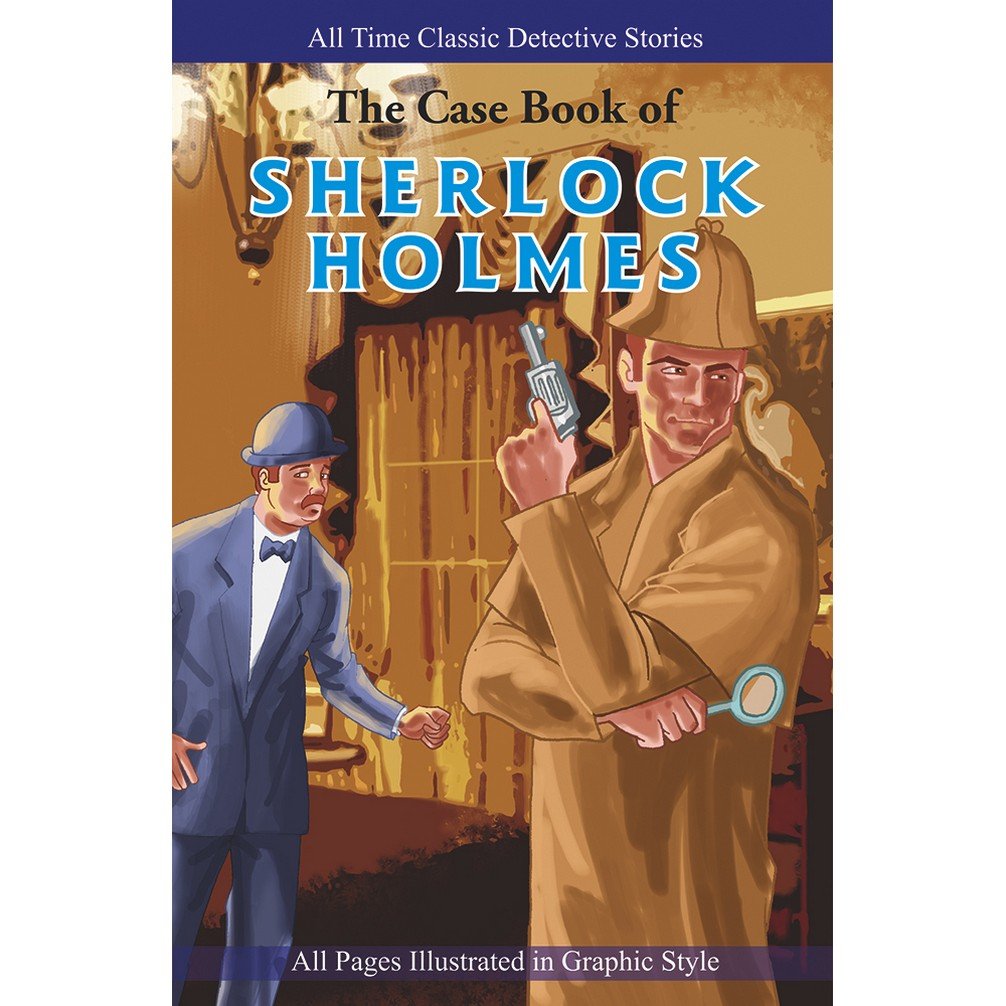The image depicts the cover of a Sherlock Holmes book titled "The Casebook of Sherlock Holmes". At the very top, there is a prominent blue bar with the words "All-Time Classic Detective Stories" written in white. Below this, the title "The Casebook of Sherlock Holmes" is split, with "the casebook of" in small black letters and "Sherlock Holmes" in larger, bright blue letters outlined in white. The background is predominantly brown and beige. To the right, there is an illustration of Sherlock Holmes, adorned in his iconic brown hat and matching coat. He holds a silver revolver in his right hand and a blue magnifying glass in his left. To the left of Sherlock Holmes stands Dr. Watson, identifiable by his blue dome hat, blue suit, and blue tie. The bottom of the cover features a translucent purple bar with white text that reads, "All Pages Illustrated in Graphic Style."